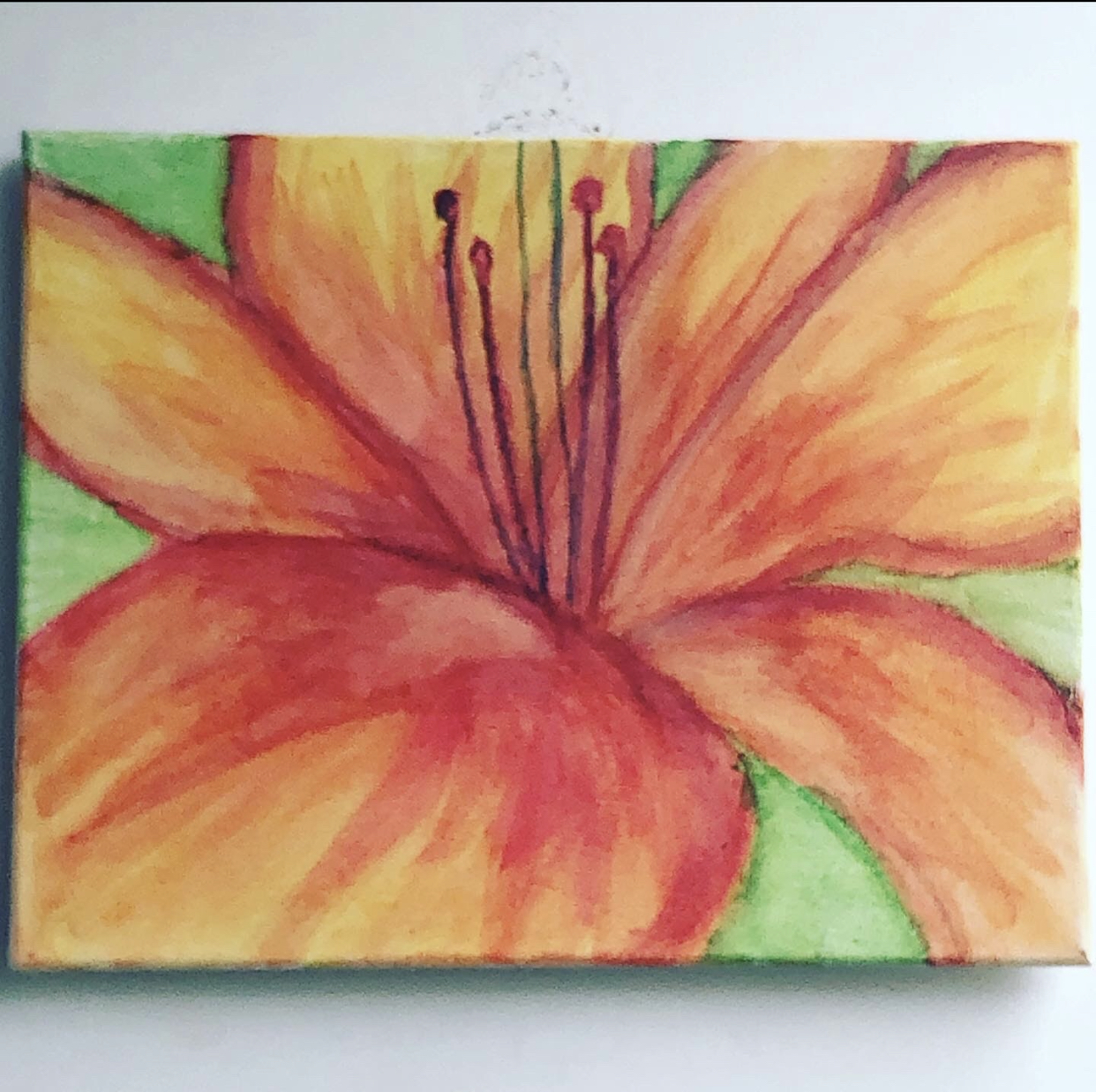This is a rectangular painting of a vibrant lily set against a lush green background. The lily's petals showcase an exquisite gradient of colors, with deep reds at the center transitioning to bright oranges and luminous yellows towards the edges. Prominently, four stamens emerge from the heart of the flower, each topped with a round, red anther. Delicate, darker lines accentuate the contours of the petals, highlighting their intricate structure and adding depth to the overall composition.